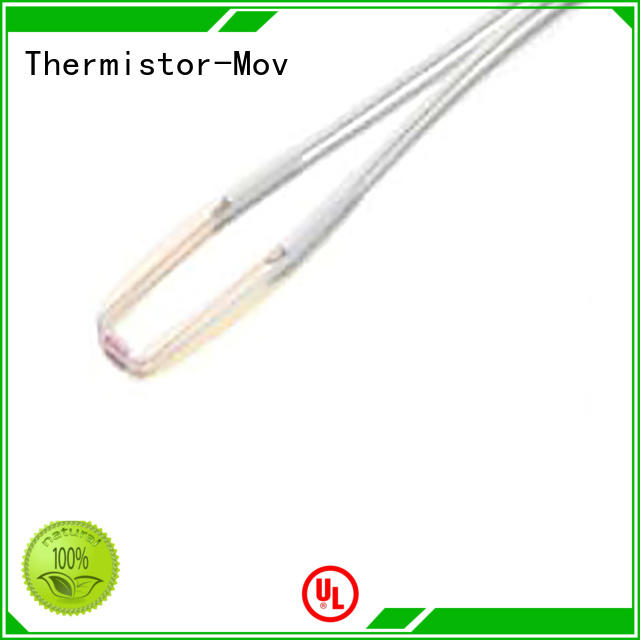The image is an advertisement for what appears to be a heating element, bordered by a green square outline. Inside, the background is white. In the upper left corner, a green bar extends about a quarter of the way across the image with the words "THERMISTOR-MOV" inside. Nearby, there's a slanted green square. From the upper right, a metallic component with two converging pieces appears; it's silver at the top, transitions to yellow as they curve outward, and then merges into a purple union at the bottom, resembling a large metal needle with an exaggerated eye.

In the center of the image, there's a prominent red circle featuring the letters "U" and "L" in white. The bottom left corner holds a green circle labeled "Natural 100%" with two leaves beneath the text, resembling an award seal. Meanwhile, the bottom right corner has another green bar extending about a quarter of the way from the right edge, next to a green square aligned to match the angle of the bar.